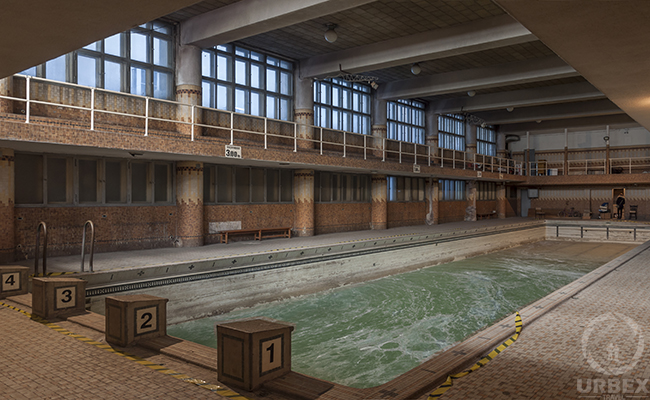This image captures an old, Olympic-sized swimming pool situated in the basement of a derelict two-story gym facility. The pool, in the process of being drained, holds a small amount of greenish water with white swirls, especially concentrated in the deep end. At the closest end toward the photographer, there are four brown wooden diving podiums labeled 1, 2, 3, and 4, encircled by yellow and black caution tape. The tan and cream-tiled floor around the pool is partially covered with a wood-tone material, possibly rug or rubber. The ground floor windows are mostly boarded up or covered, while the second-floor windows are open, allowing light to cascade through. Cylinder poles stretch from the ground to the top floor, supporting a metal balcony with a white banister that rings the upper level. Above, silver beams and round white globe lights (currently off) adorn the ceiling. In the bottom right corner of the image, there is a notable circle featuring the word "URBEX". Three individuals are visible at the far end of the pool: one standing and two seated, seemingly observing the scene.